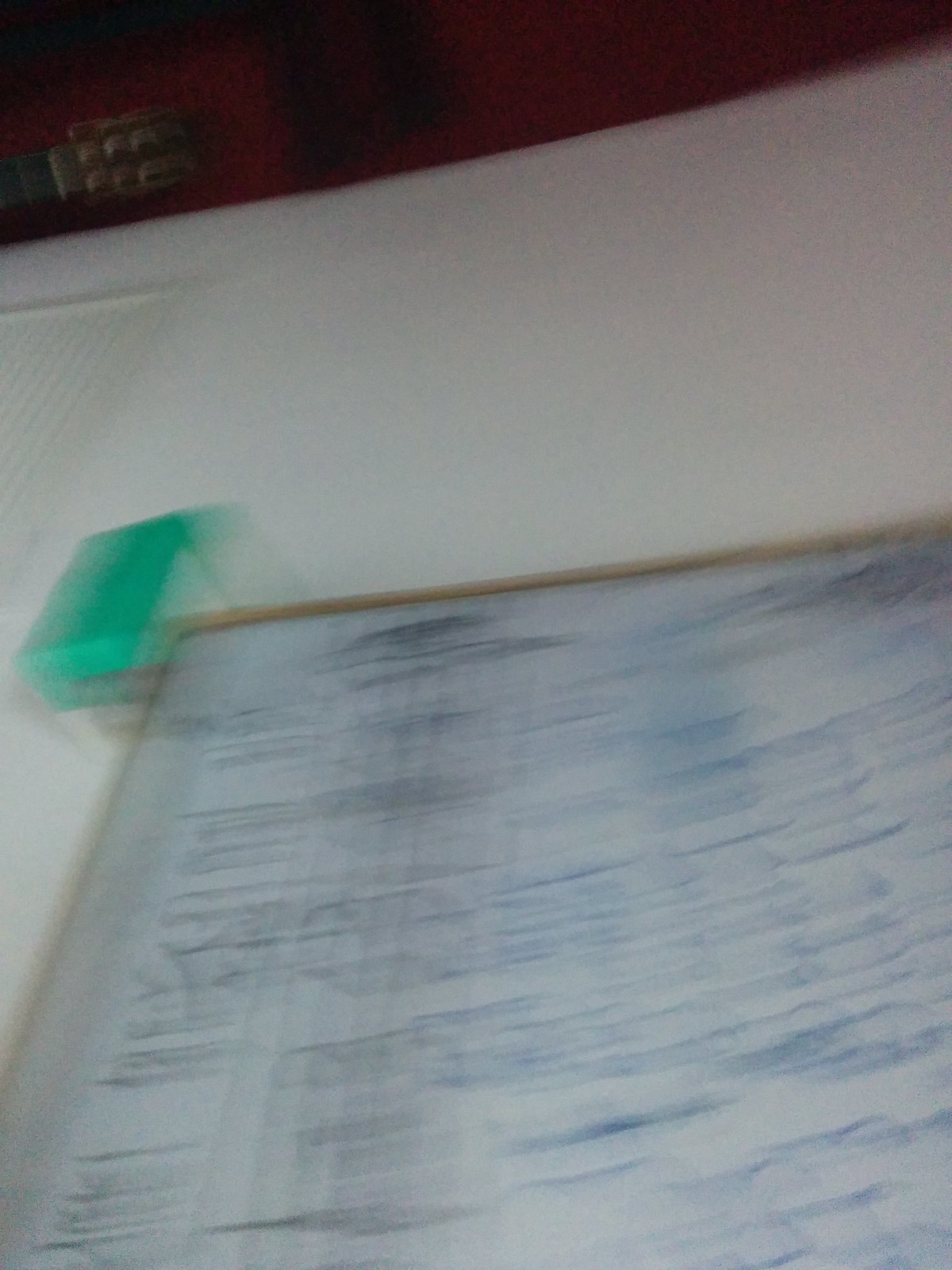This extremely blurry photograph depicts an indoor scene captured in low light without a flash. The top portion of the image shows what appears to be a dark red or brown paneled wall with some black highlights. Notably, a sideways guitar neck is visible in the top left corner, indicating the photograph may be rotated 90 degrees. Below this, a white surface—likely a whiteboard with a pale wooden frame—is seen against a white wall or possibly a white sofa. The board is heavily scribbled with indistinguishable markings, blue writing on the right, and black writing including vertical lines on the left, suggestive of musical notes and clefs. Additionally, there is a bright greenish-blue container attached to the top left corner of the whiteboard. The overall blurred nature of the image and the mixed accounts suggest the scene might include an artistic or musical setup.